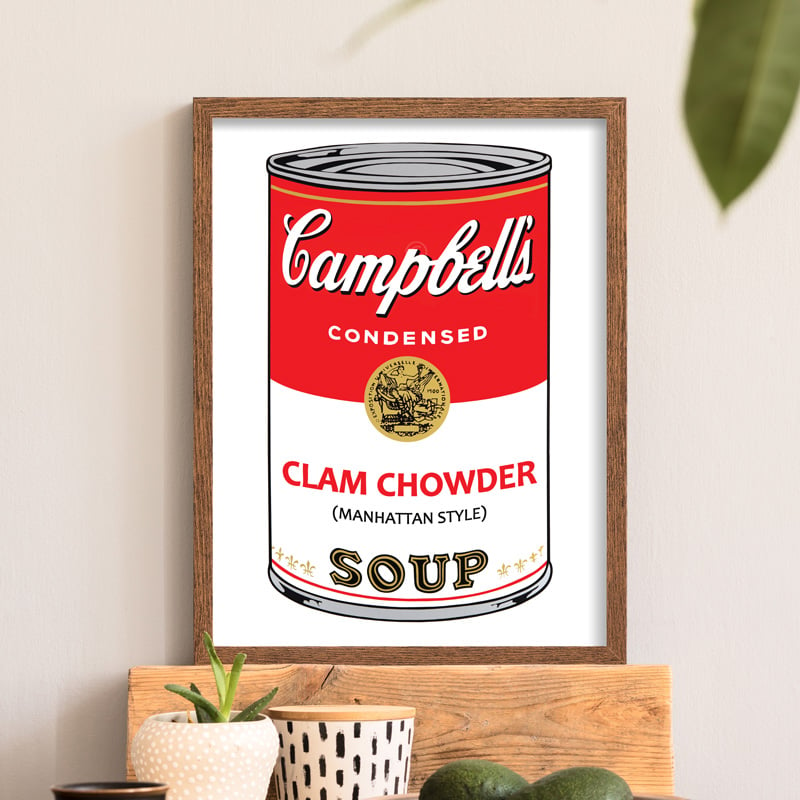The horizontally aligned, rectangular photograph captures an indoor scene featuring a framed artwork prominently displayed. The main focal point is a painting or print assumed to be a piece by Andy Warhol from the 1960s or 70s. This artwork displays a Campbell's condensed clam chowder soup can, enclosed in a dark brown wooden frame that could be either real or faux wood. The frame appears slightly wider on the sides, and the photo might be slightly distorted making the frame look gently squished.

The Campbell's soup can depicted in the artwork is straightforwardly detailed. The can has a red upper half and a white lower half, separated by a gold band running around its circumference. The top is depicted with a silver metal rim and the bottom edge includes a similar silver detail. "Campbell's" is written in bold, cursive letters at the top of the can with "condensed" centered directly underneath in smaller uppercase letters. The can's middle section features a gold or tan circle with a finely detailed, possibly landscape-style black drawing, suggesting a 1920s aesthetic. Below this circle, in larger red uppercase letters, it says "clam chowder," and under that, in black uppercase text in parentheses, it reads "Manhattan style". The word "soup" is at the bottom in a classic font, highlighted by tan and black stripes, accompanied by three tan stars on the left and four on the right. 

The framed artwork rests horizontally on what appears to be a polished wooden stand, likened to a 2x4 with visible wood grain. In the foreground, two green avocados lie on their sides, partially visible. Next to them, there's a bowl with a tan wooden lid; the bowl itself is white with black rectangular spots. To its left is another bowl, predominantly tan with white spots, containing an aloe vera plant with about six sharp, triangular leaves. Below this bowl, only the rim of a smaller black bowl is visible. The background of the photograph is a white wall, casting shadows near the left and right edges of the frame. Additionally, the upper right portion of the image contains a leaf from a tropical plant, angular and wide, with faded veins running through it.